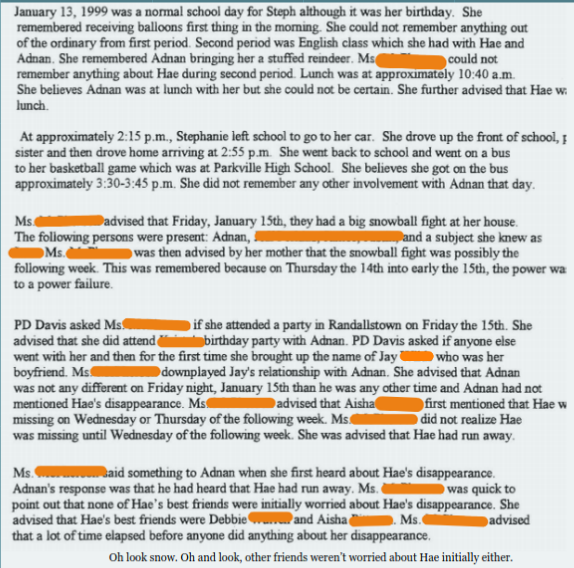**Caption:**

The image features a considerable amount of text written in black on a light gray background. The text elaborates on a series of events and statements made by a girl named Stephanie regarding January 13th, 1999, which was her birthday and a usual school day for her.

Steph recalls receiving balloons in the morning and describes her routine through various periods of the school day. She particularly remembers Adam, a fellow student, bringing her a stuffed reindeer during English class in second period but does not recall any specific details about another student named Hay. During lunch at approximately 10:40 a.m., Steph believes Adnan was present but isn’t certain. The text is partially cut off mentioning Hay at lunch.

Details of Steph's afternoon include her leaving school at 2:15 p.m., driving up to the front of the school, and then heading home, arriving at 2:55 p.m. She later returned to the school to take a bus to her basketball game at Parkville High School, estimating the bus departure between 3:30 and 3:45 p.m. Steph does not recall any further interactions with Adnan that day.

Further into the narrative, Steph talks about an event held at her house on Friday, January 15th, where a group of people, including Adnan, participated in a snowball fight. However, her mother later suggests this event could have occurred the following week, which was notable due to a power failure on January 14th or 15th.

Additionally, Steph mentions attending a birthday party in Randallstown on the same night, the 15th, with Adnan. When asked by PD Davis, she also mentions Jay for the first time, who was noted as her boyfriend. Steph describes that Adnan behaved no differently that night and never mentioned Hay’s disappearance.

The text further reveals that Aisha was the first person to inform Stephanie about Hay being missing, which was either on Wednesday or Thursday of the following week. Initially, no one seemed particularly worried, as they assumed Hay had run away. Steph highlights that none of Hay’s best friends, namely Debbie and Aisha, expressed immediate concern. She emphasizes that a significant amount of time passed before any serious actions were taken regarding Hay’s disappearance.

The bottom of the text, written in a different font, states, "oh look snow and oh and look other friends weren’t worried about Hay initially either."